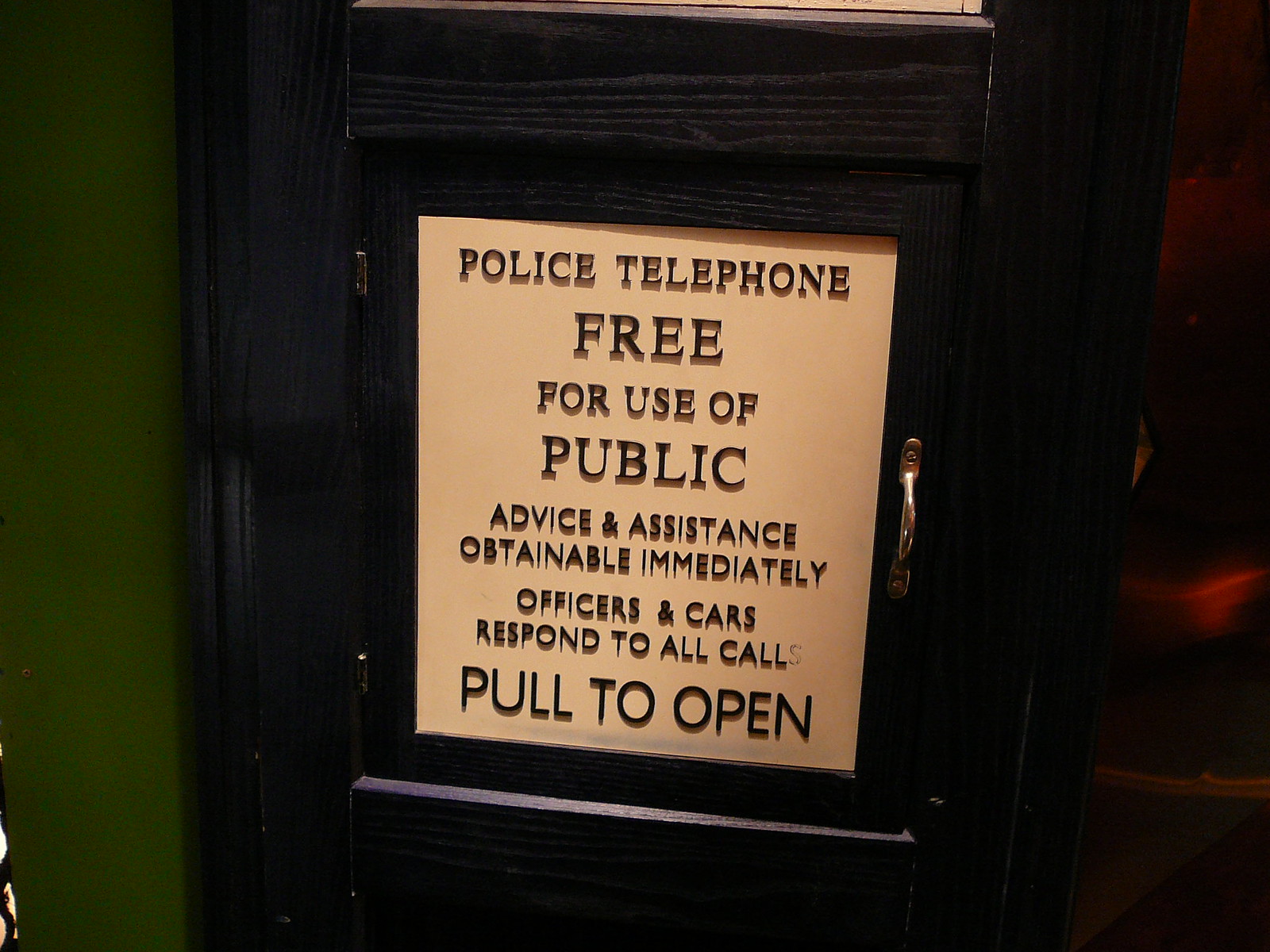This image features a close-up of a panel on a traditional British police box, resembling the iconic TARDIS from Doctor Who. The box is painted blue and made of wood, and prominently features a white informational panel with black text. The text reads: "POLICE TELEPHONE FREE FOR USE OF PUBLIC. ADVICE AND ASSISTANCE OBTAINABLE IMMEDIATELY. OFFICERS AND CARS RESPOND TO ALL CALLS. PULL TO OPEN." Notably, the letter 'S' in "ASSISTANCE" appears scratched, nearly removed. To the right of this panel is a silver, chrome-like handle, giving the panel the appearance of a door. The handle is metallic and robust, suggesting functionality. The surrounding environment is dimly lit, making it difficult to discern details clearly. However, parts of a green wall are visible to the left, while the right side reveals a brown wooden section, possibly a doorway. The text on the panel is entirely uppercase, contributing to the authentic look of this iconic police public call box.